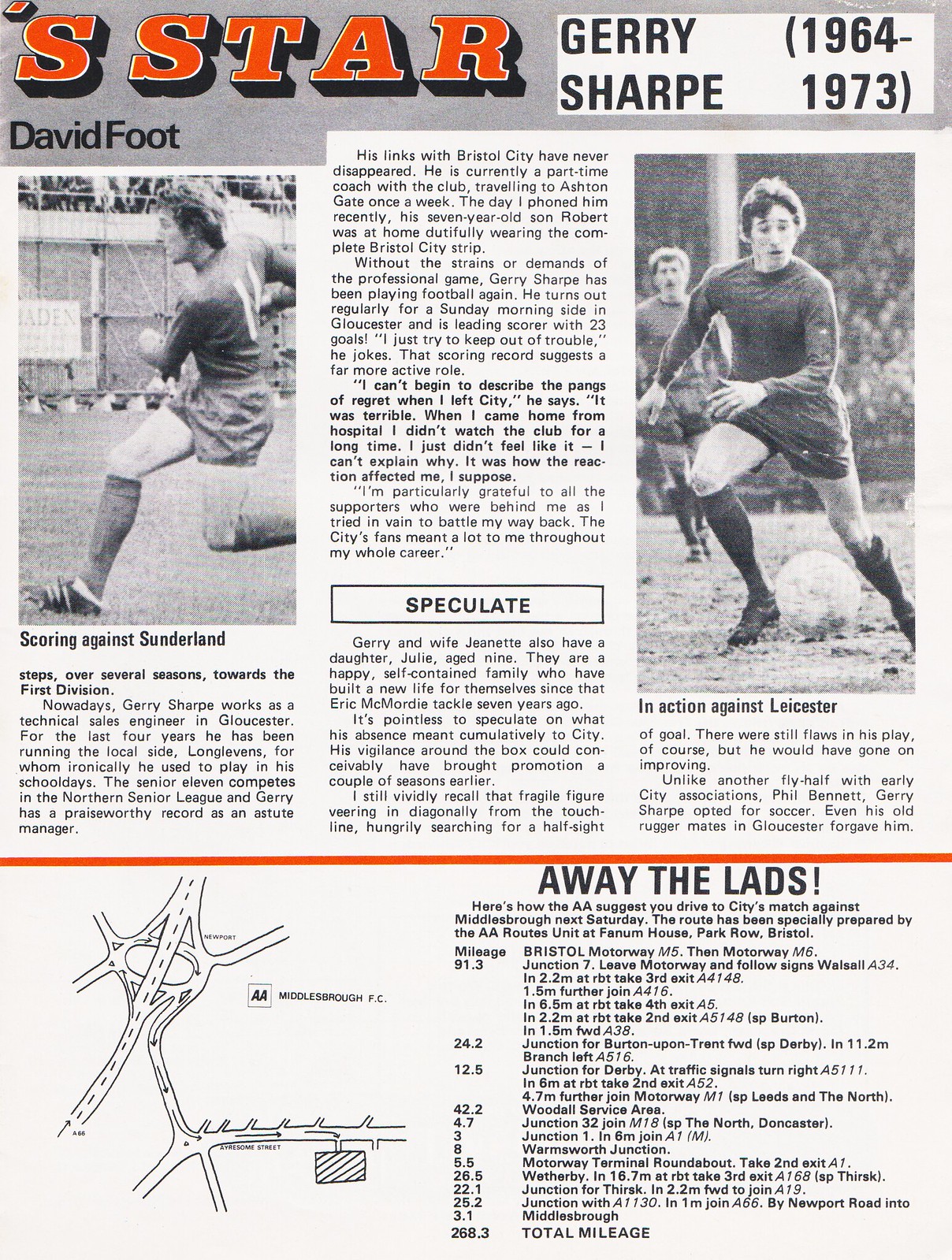The image is a vertically aligned rectangular clipping from a newspaper, primarily in black and white with prominent orange accents. The headline at the top reads "S STAR" in large, orange, block letters. Below it, in black text, is the name "David Foote." To the right, within a white rectangle, "Jerry Sharp (1964-1973)" is written in black text.

The upper half of the clipping features what appears to be an obituary or profile, with three columns of text. The left and right columns each contain black-and-white photos of soccer players in action. The left photo's caption reads "David Foote scoring against Sunderland," while the right photo's caption states "in action against Leicester." Both players are depicted in their dark-colored soccer uniforms, with noticeable movement captured on the field.

Beneath this section, a thick, horizontal orange line separates the upper half from the lower half. The lower half is headlined "AWAY THE LADS" in all-black capital letters, emphasizing directions to a stadium match. To the left is a black-and-white map illustrating the suggested driving route to the stadium, with columns detailing mileage and Bristol Motorway directions. The entire clipping appears to be a nostalgic tribute, combining personal anecdotes about Jerry Sharp and practical information for attending a soccer match.